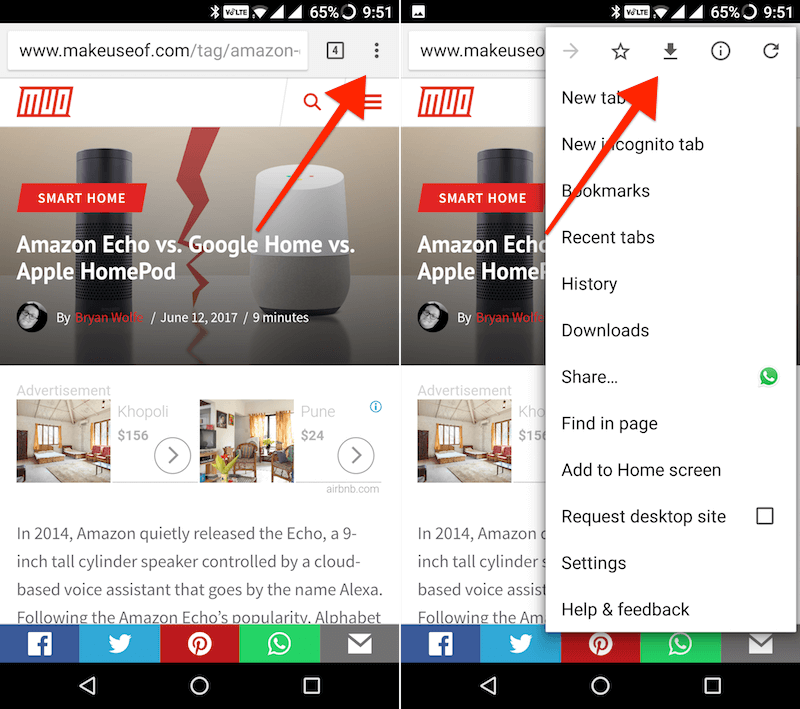This image is a photo collage comprising two nearly identical screenshots taken from a mobile phone, likely as part of a tutorial walkthrough. Both screenshots feature the standard elements seen on a mobile device: a black status bar at the top displaying the Bluetooth symbol, LTE indicator, Wi-Fi signal strength, cellular connection, a battery level at 65%, and the time, which reads 9:51.

Directly beneath the status bar in both images is the address bar showing the URL www.makeuseof.com/tag/Amazon, truncated at the end. Below the address bar, the webpage header reads "MUO" and features an image of an Amazon Echo device and a Google Home, alongside the article's title – "Smart Home: Amazon Echo vs. Google Home vs. Apple HomePod" authored by Brian Wolf, dated June 12th, 2017, with a reading time of 9 minutes.

The bottom section of both screenshots displays various sharing options, including Facebook, Twitter, Pinterest, WhatsApp, and email. A notable addition is the red arrow in each screenshot, drawing attention to specific features. In the first screenshot, the red arrow points to the three vertical dots next to the search bar, indicating the options or menu area. In the second screenshot, the red arrow focuses on the downward-facing arrow icon, representing the download option.